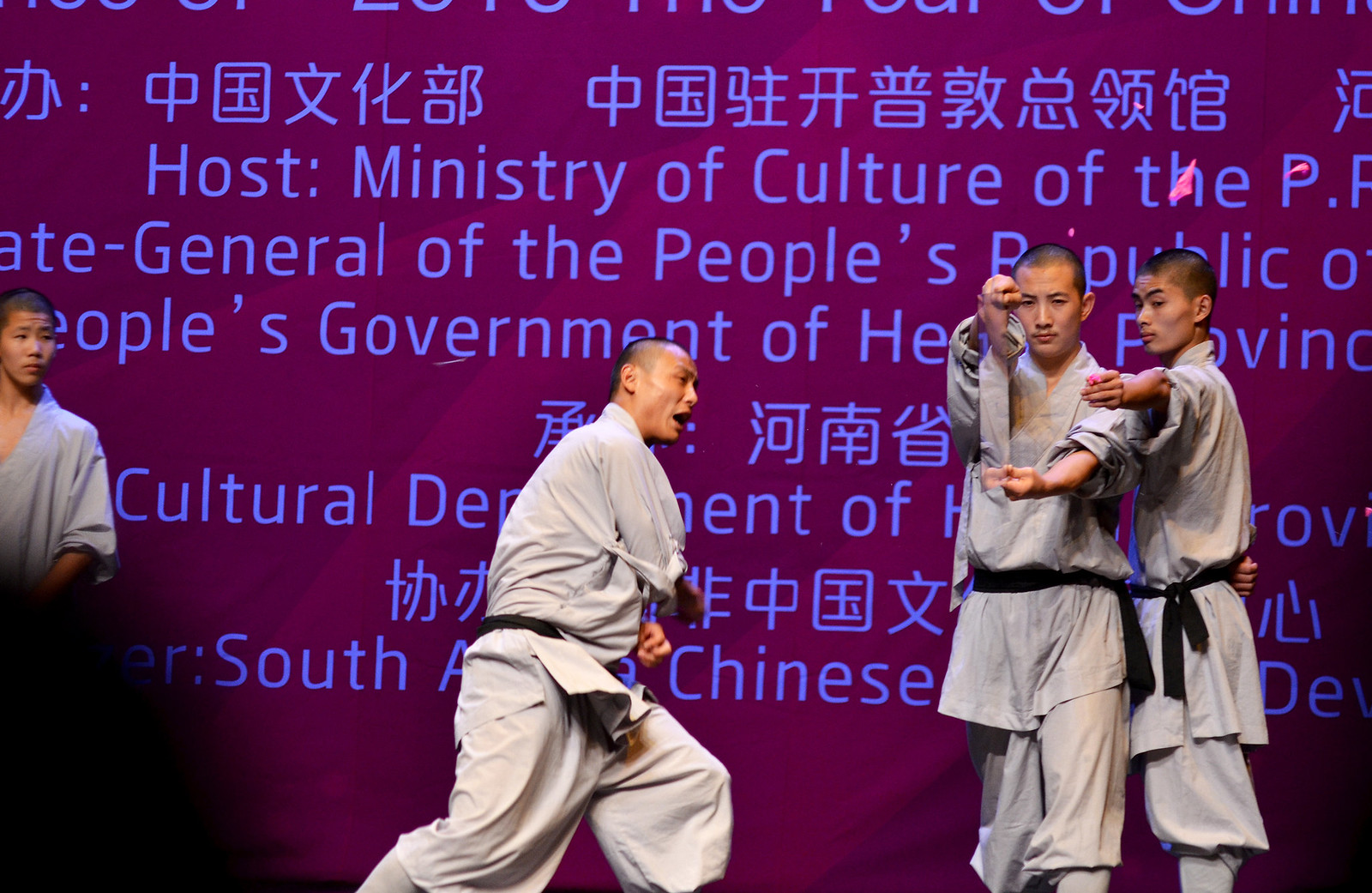This photograph captures a dynamic moment during a martial arts exhibition staged on a platform. Centered in the image is a man dressed in a light gray karate uniform with a black belt, appearing to have just struck a board out of a younger man's hands. This younger man stands to the right of the central figure, also attired in a matching gray karate robe with a black belt, holding a reflective glass pane or board, firmly gripped with both hands near his chest and face. Supporting him from behind, another man extends one arm to buttress the glass or board. All three individuals have short black hair and appear to be of Asian descent. To the far left, partially cropped out, is another man dressed similarly, observing the action. The backdrop features a large, dark red banner with partially obscured light blue text, containing phrases such as "Host, Ministry of Culture of the People's Republic of" and "People's Government of." Additionally, a shadow or silhouetted head of a spectator is visible at the bottom left corner, indicating a live audience is present.